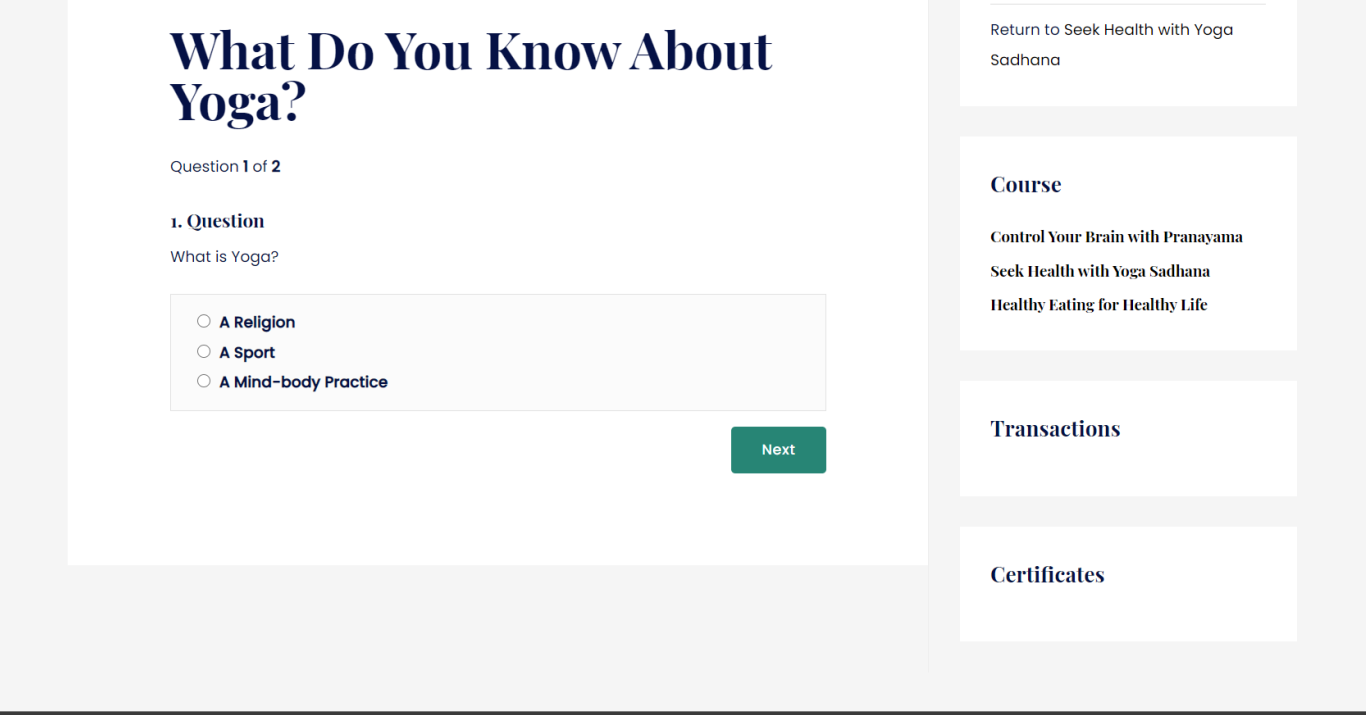This website screenshot centers around a quiz designed to gauge knowledge about yoga. The backdrop is an off-white hue, contrasting with white boxes that contain black text. In the center of the page is a prominent question within a white box, asking "What do you know about yoga? Question one of two." The first question presented is "What is yoga?" with three selectable options: a religion, a sport, and a mind-body practice. A turquoise button labeled "Next" is positioned at the bottom right of this box.

On the right side of the screenshot, four vertically stacked white boxes feature additional black text. The top box reads "Return to seek health with yoga sadhana." Below it, the second box says "Course: Control your brain with pranayama. Seek health with yoga sadhana. Healthy eating for healthy life." The third box is labeled "Transactions," and the fourth box says "Certificates."